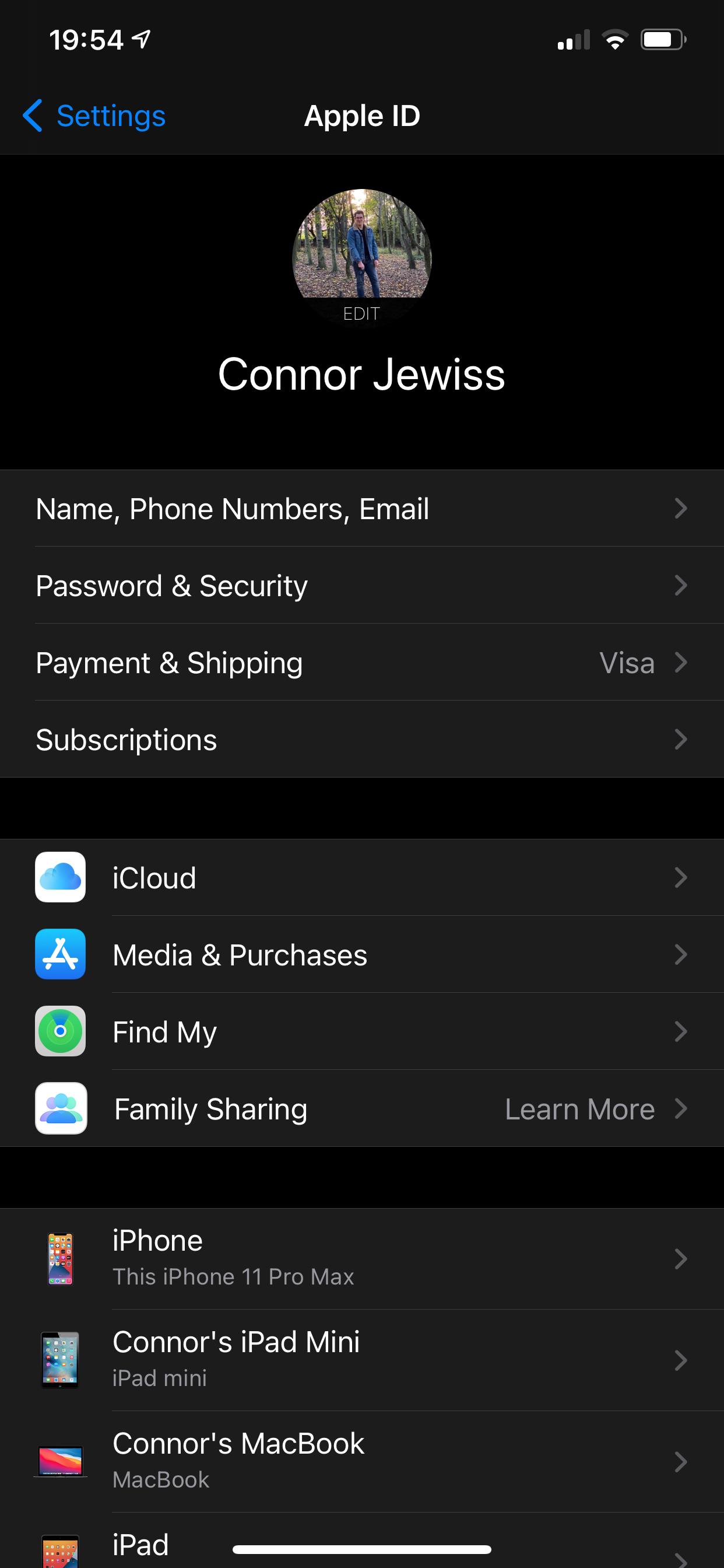This is a detailed caption to describe the image:

The screenshot depicts the Apple ID settings page of an iOS device, specifically an iPhone 11 Pro Max, as indicated at the bottom of the screen. The interface features a predominantly black background, suggesting the use of Night Mode. At the top left, the time is displayed as 19:54, accompanied by a location arrow, implying that GPS services are active. Below the time is a blue-colored "Settings" label and a back button pointing to the left.

Centered at the top is the header "Apple ID", flanked on the right by network indicators showing 2 out of 4 signal bars and a Wi-Fi signal strength of 2 out of 3. The battery icon suggests approximately 85% charge, despite the absence of an exact percentage.

Underneath the "Apple ID" header, there is a circular profile image of the phone's owner, Connor Jewiss (spelled J-E-W-I-S-S). He is depicted in a blue jacket in a forested area, possibly around 5 PM, based on the lighting and shadows. His name is displayed below his picture, followed by sections labeled "Name, Phone Numbers, Email", "Password and Security", "Payment & Shipping", and "Subscriptions".

Further down, four icons are listed in rows under the categories: iCloud, Media & Purchases, Find My, and Family Sharing. Each has a corresponding "Learn More" link next to it.

At the bottom, the devices associated with Connor's Apple ID are listed, including "This iPhone 11 Pro Max", "Connor's iPad mini", and "Connor's MacBook".

Overall, the screenshot provides a comprehensive view of the Apple ID settings page, highlighting various profile details and device connections managed by Connor Jewiss.